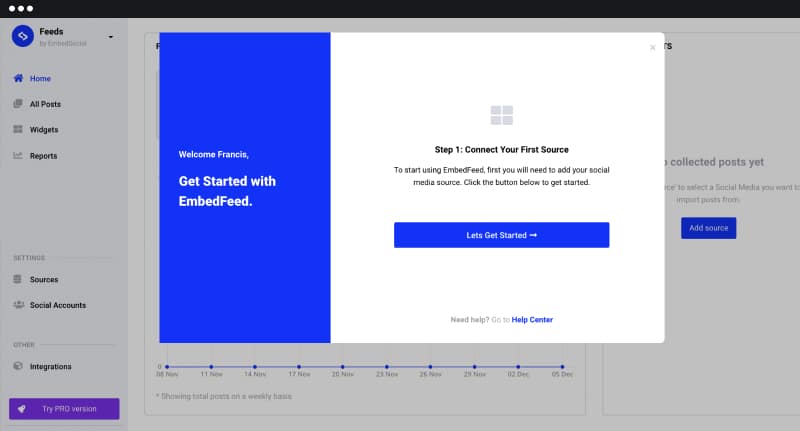In the image, a website interface is displayed, featuring a sidebar on the left and a main content area in the center. The sidebar has a light grey background with various menu options. The first option, "Home," is highlighted in blue. Other options listed below it include "All Posts," "Widgets," and "Reports." Towards the bottom of the sidebar, there are additional options such as "Sources," "Social Account," "Integrations," and a purple button labeled "Try ProVision." The top of the sidebar features a section named, "Feeds by Embedded Social," accompanied by a blue icon with white arrows.

The main content area of the page is divided into two sections, each with different backgrounds. On the left half, a blue section welcomes the user with the text, "Welcome Francis, get started with EmbedFeed," written in white font. On the right half of the page, the background is white with instructions labeled as "Step 1: Connect to your first source." Below this, it explains that to start using EmbedFeed, the user must add their social media source by clicking a blue button that says "Let's get started." Beneath this, there is a prompt saying "Need help? Go to help center," with "Help Center" highlighted in blue.

Behind the main content, a semi-transparent graph with colored segments is visible, though it lacks any numerical values. Additionally, towards the right side of the image, there is another blue button labeled "Add Source."